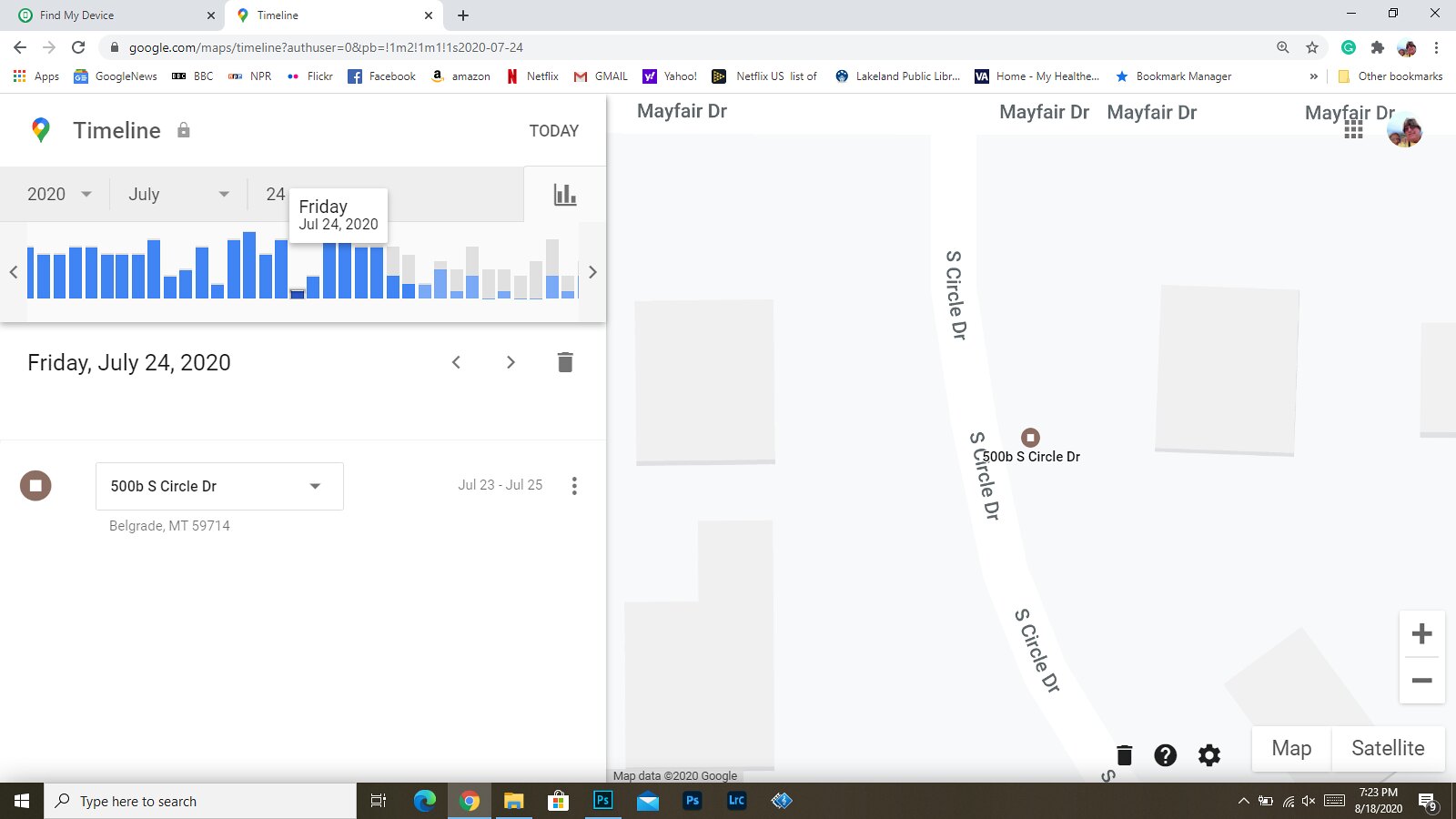This image is a detailed screenshot from Google Maps, opened in Google Chrome. The map on the right side prominently features the Mayfair Drive area, with South Circle Drive extending southward from Mayfair Drive. The user is specifically searching for 500 B South Circle Drive. In the upper left corner of the screenshot, a timeline is visible, indicating past activity or locations. The interface indicates that it is possible to switch to a satellite view of the map. Another browser tab, not currently in focus, is labeled "Find My Device," suggesting the user is attempting to locate a lost device that may be somewhere along South Circle Drive.